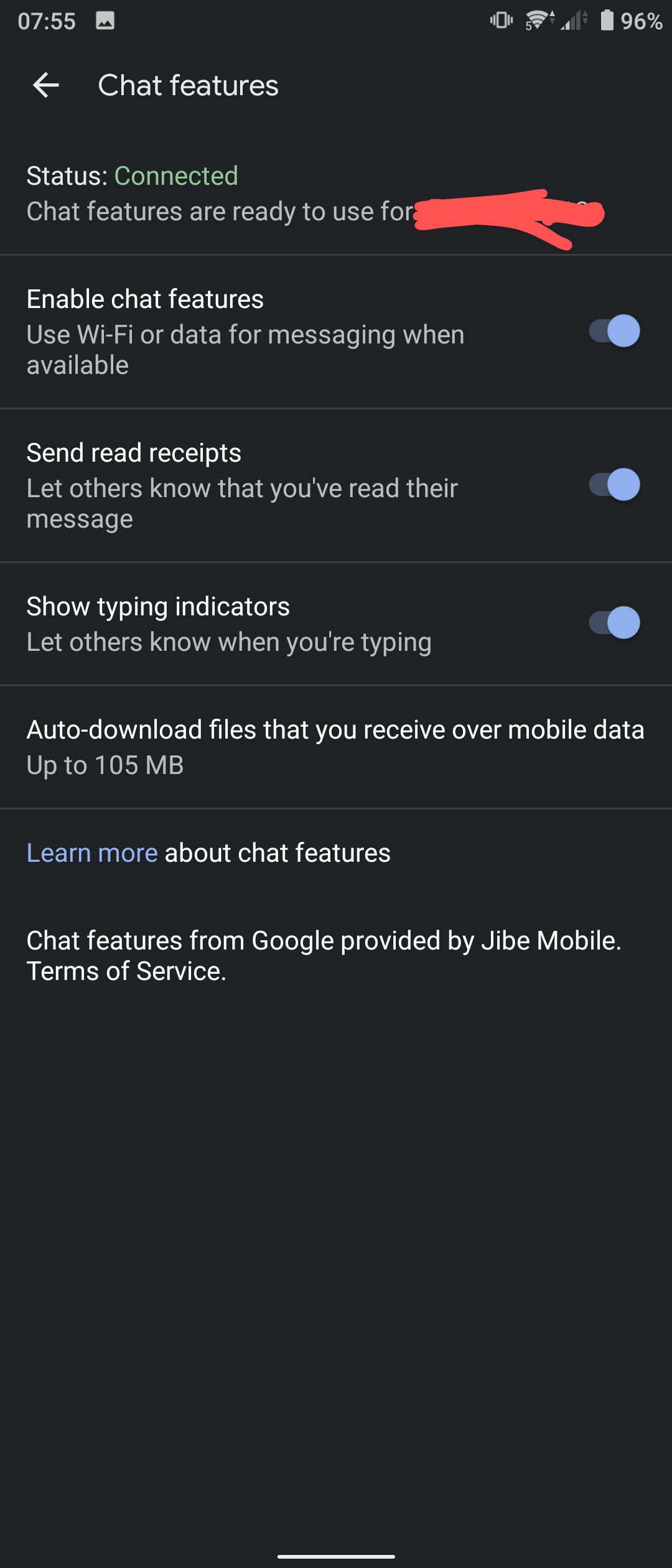Screenshot of an iPhone in landscape mode displaying the chat features settings:

- The screenshot shows an iPhone in landscape orientation.
- The time is displayed on the left-hand side of the status bar at 10:55.
- The phone is set to vibrate mode.
- Wi-Fi is enabled, and the device has two bars of signal strength with a battery level at 96%.
- The interface has a black background with white text.
- At the top of the screen, there is a back button labeled "Chat" indicating navigation to chat features.
- The status of chat features is "Connected" in green.
- Below, it says "Chat features are ready to use" followed by a red-crossed-out note and an option to "Enable chat features."
- The option "Use Wi-Fi for data managing when available" is checked.
- There are toggle buttons for:
  - "Send read receipts" (enabled, allowing others to know when messages are read).
  - "Show typing indicators" (enabled, allowing others to see when the user is typing).
- The auto-download feature for files over mobile data is set with a limit up to "105 MB."
- A blue link for "Learn more" followed by text about chat features provided by Google and Jiba Mobile's terms of service.
- The rest of the background fades to black towards the bottom of the screen.

This detailed caption describes the various elements visible in the screenshot including the device settings, status indicators, and chat features configuration.